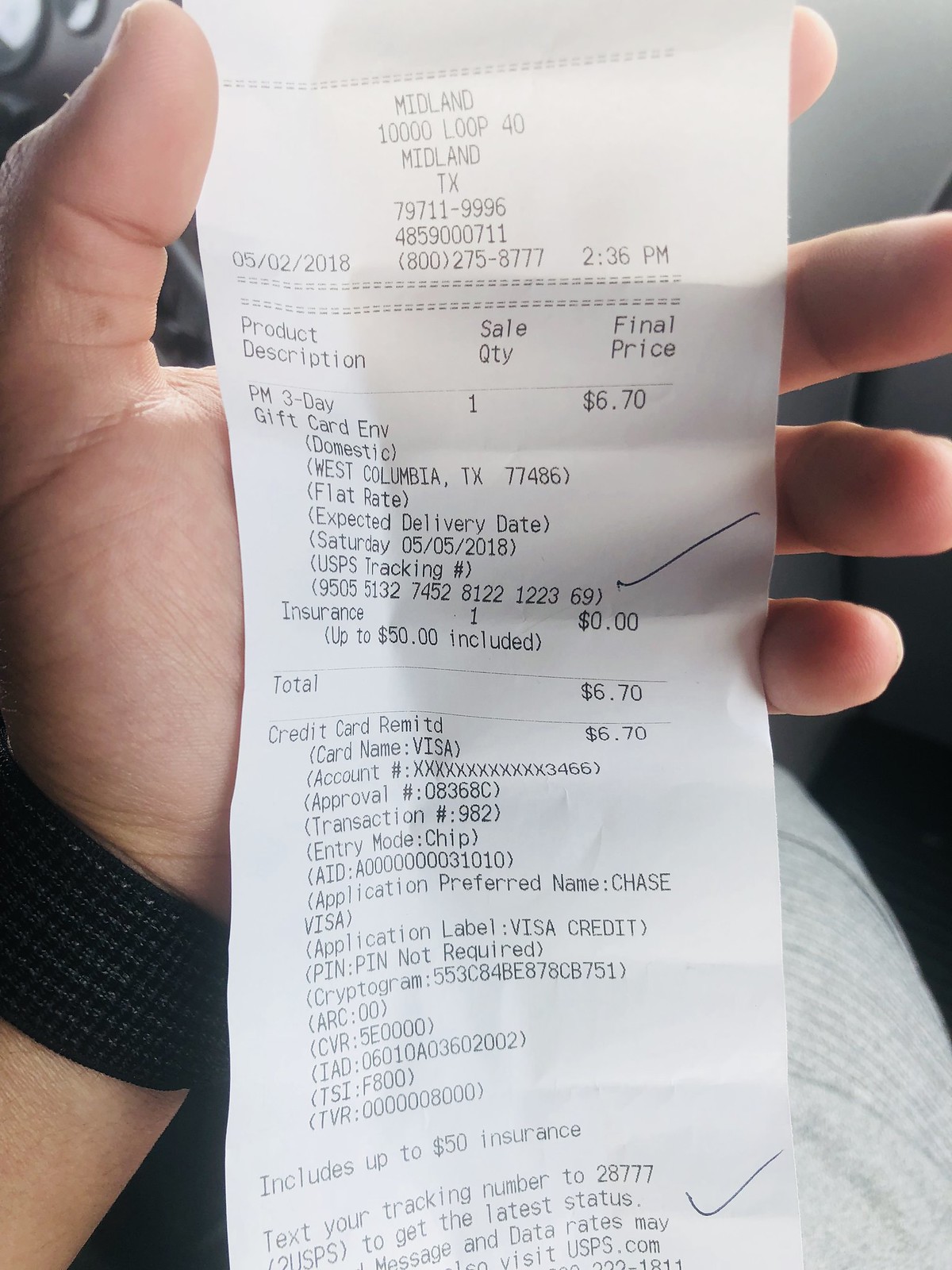The image depicts a close-up of a man’s hand holding a long, white thermal receipt against a gray background. The man is wearing a textured black wristband, possibly a watch. The receipt prominently displays the heading "Midland" followed by the address "10,000 Loop 40, Midland, Texas, 79711-996." Dated May 2, 2018, at 2:36 PM, the receipt includes a phone number, 800-275-8777. It details the purchase of a "gift card envelope" sent via PM 3-day flat rate, with a sale quantity of one at a price of $6.70. Payment was made using a Visa credit card. The receipt also mentions that it includes up to $50 of insurance and provides tracking number details, although it cuts off the specific instructions for tracking. An additional detail includes a checked line on the right side of the receipt, suggesting a verification mark.